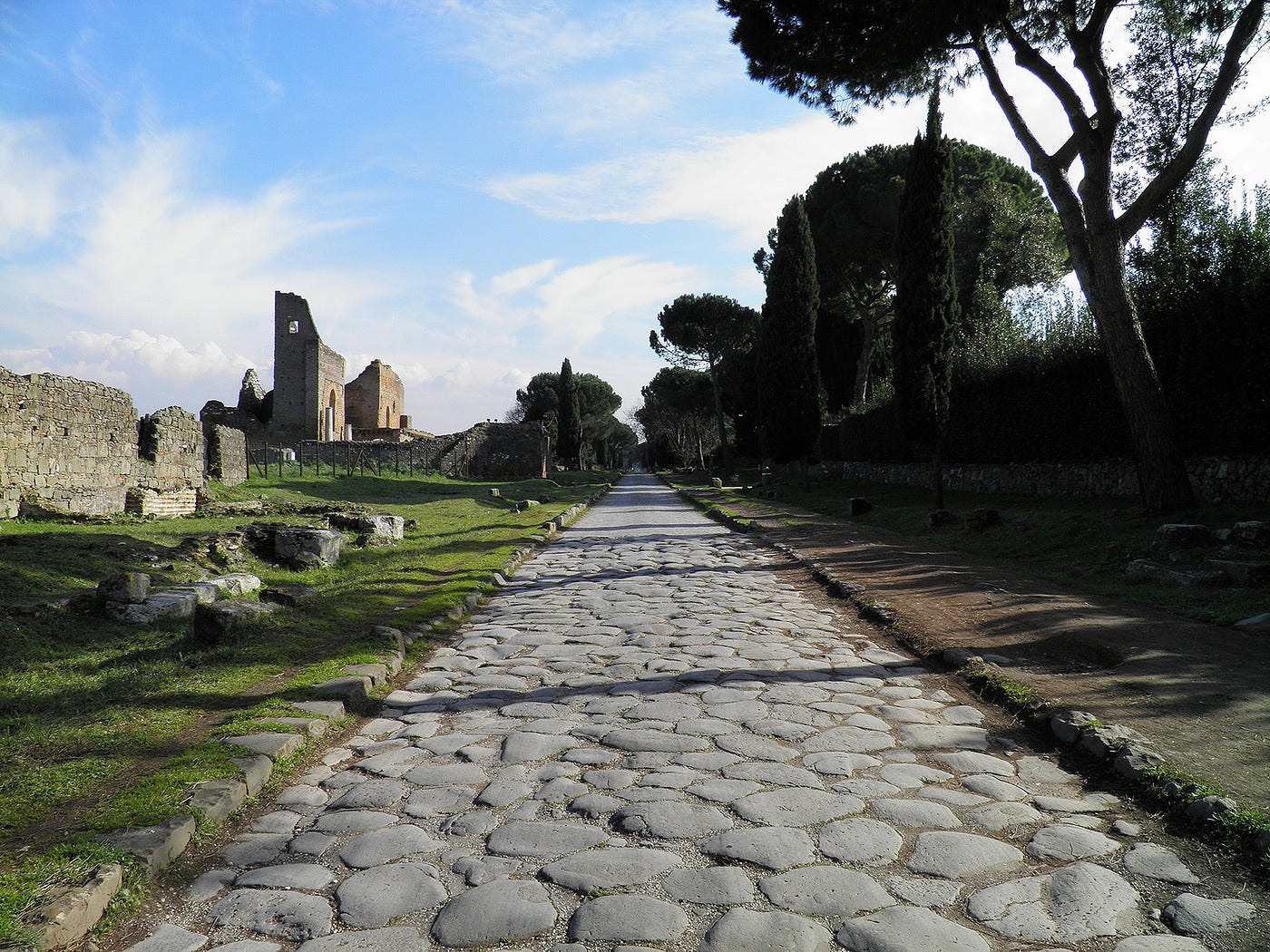This photograph captures a serene and ancient cobblestone pathway, stretching far into the distance, evoking a sense of historical depth. The path, characterized by its gray stones, conjures the architectural traditions of the late 17th to early 18th centuries, suggesting its location might be in Europe or the United Kingdom. On the right side of this pathway, a well-manicured row of trees forms a natural border. These trees exhibit a carefully tended appearance, with some pruned into perfect dome shapes, achieved through diligent shearing. A dirt path runs parallel to the cobblestone road, shaded by tall trees with thick canopies of green leaves that cast intricate shadows on the ground. To the left of the pathway, a grassy lawn unfolds, leading up to the ruins of an old stone structure resembling a fort, notable for its partially decayed walls and tall, arched doorways. Rising in the background, the remnants of an ancient stone church punctuate the horizon under a bright blue sky with puffy white clouds, enhancing the picturesque and timeless quality of the scene. The image is devoid of any foot traffic, adding to its tranquil and undisturbed atmosphere.